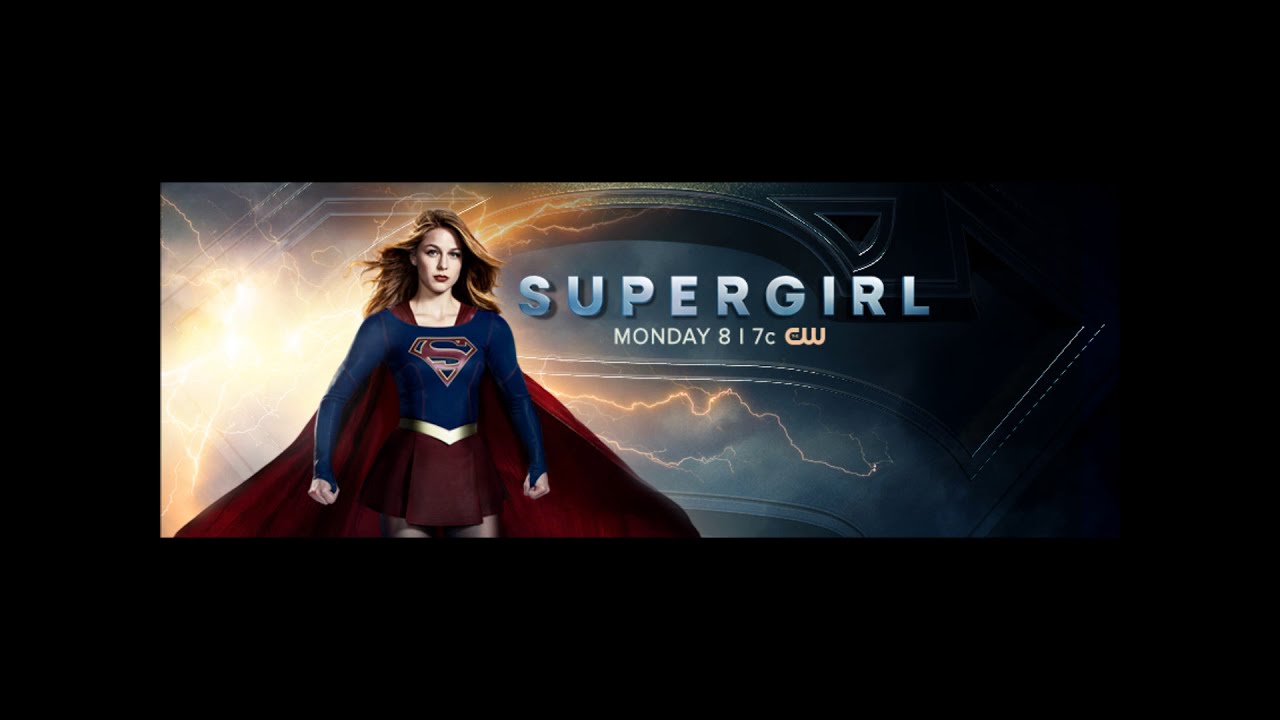The image is a promotional graphic for the television show Supergirl, featuring a rectangular, landscape-oriented format with a thick black border. Dominating the center of the image is a striking depiction of Supergirl, captured from her thighs to the top of her head. She stands with her hands on her hips, exuding confidence. Her brown hair flows behind her shoulders and down her back, while she wears the iconic Supergirl costume: a blue, long-sleeved top adorned with the red and gold 'S' emblem on her chest, a red skirt with a gold belt, and a red cape billowing out behind her.

The background features a dynamic and electrifying scene with a sky crackling with lightning bolts and a subtle, translucent Superman emblem illuminated by the lightning. Beneath Supergirl, the title "SUPERGIRL" is prominently displayed in metallic silver and blue text, enhancing the dramatic effect. Below this, the broadcast information is provided: "Monday, 8-7c" on the CW network. The composite elements create a vivid and compelling promotional image that effectively conveys the superhero’s power and the show's airing details.